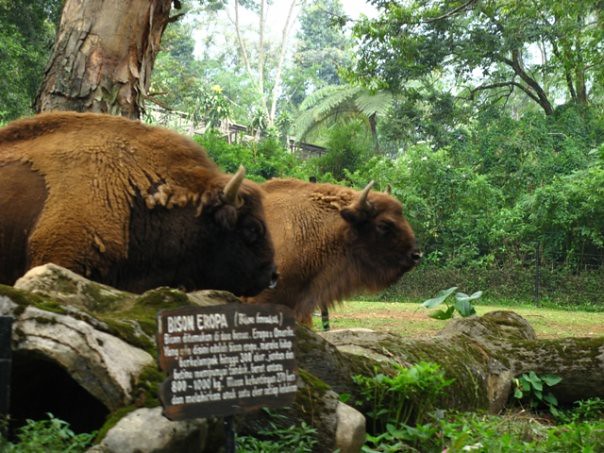The photograph captures a zoo or natural history museum exhibit featuring two realistic bison figures with brown fur and horns, identified as "Bison Europa." These bison stand amidst a backdrop of trees and grass, partially obscured by a fallen tree trunk in the foreground. To the left of the image, there is a dark brown, rough wooden plaque displaying some information, but the text is largely unreadable due to blurriness, except for the visible weight range "800 to 1,000 kilograms." This detailed setting suggests a carefully curated exhibit aimed at providing an educational glimpse into the natural habitat of the European bison.